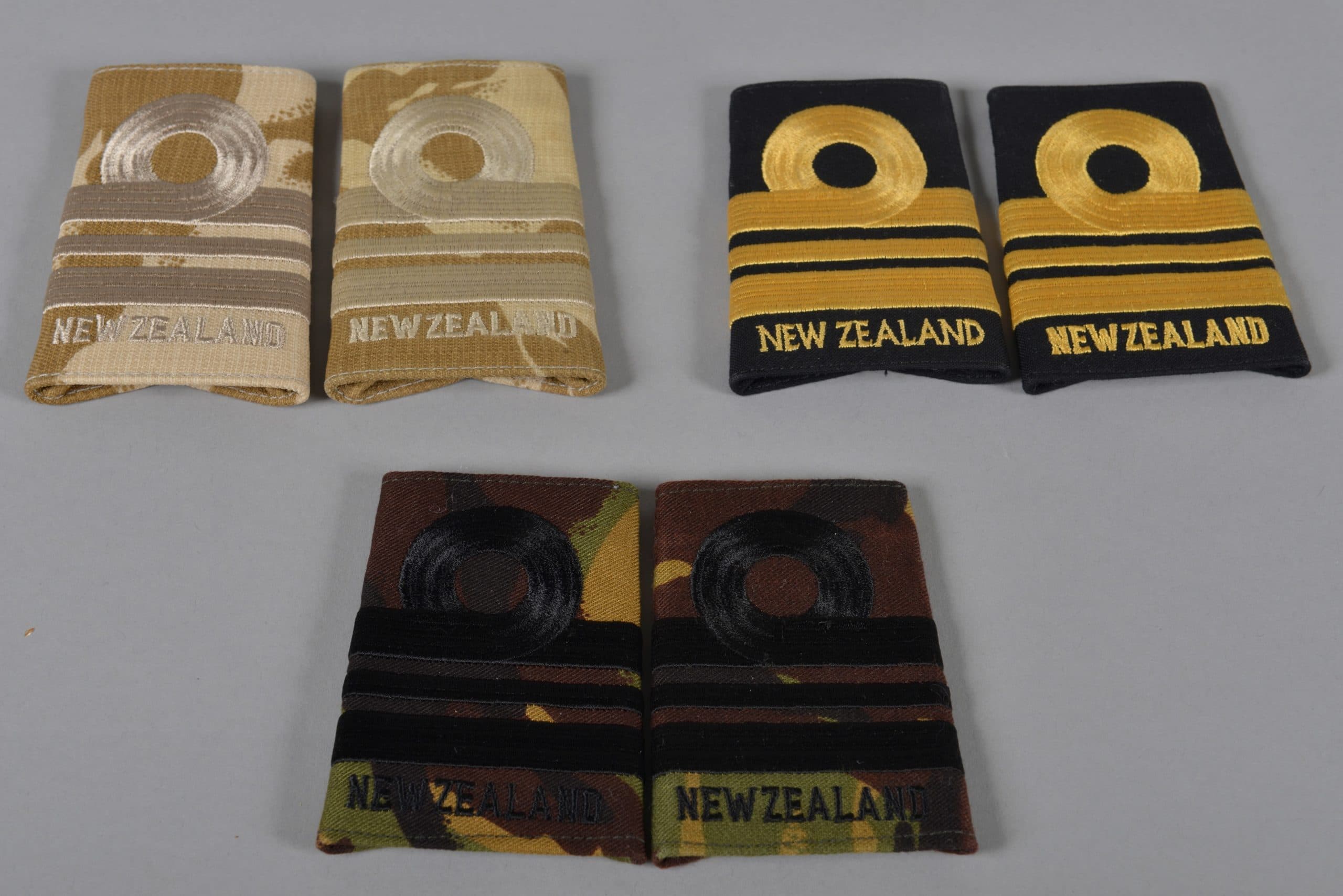The photo features three distinct sets of military patches arranged on a gray table. Each patch prominently displays a circular emblem at the top, followed by three thick lines, and finishes with the text "New Zealand" at the bottom. 

- The top left set comprises patches in light tan and brown hues, featuring a silver circle and silver lettering.
- The top right set consists of black patches adorned with gold circles and gold lettering.
- The bottom middle set showcases patches with a camouflage background of tan, light green, and brown, together with a black circle and black lettering.

All patches are uniformly designed, displaying the New Zealand insignia, and positioned neatly within their respective groups.